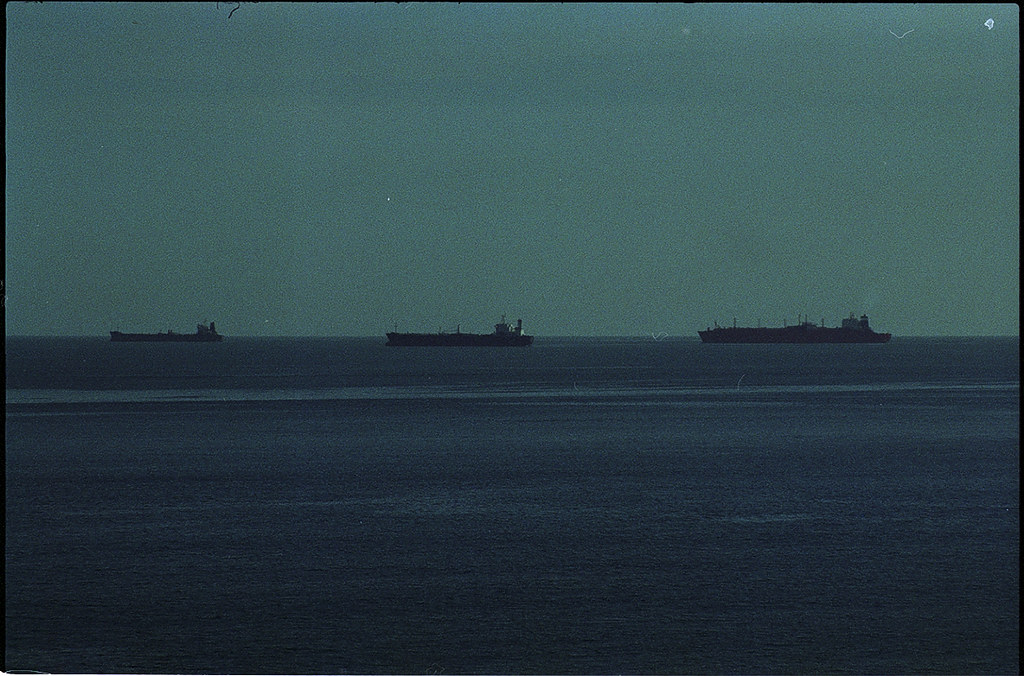In this dark and grainy nighttime image, we see a tranquil, deep blue expanse of water, possibly an ocean or sea, meeting a very dark turquoise sky. The calm water, with subtle ripples and streaks of lighter color, stretches out into the distance under a sky that features occasional white specks, perhaps stars. Dominating the scene are three large, black ships, aligned in a row. These vessels, which could be military ships, cargo ships, or oil tankers, differ in shape and size but share similar characteristics. They have flat decks and tall structures resembling watchtowers or smokestacks, positioned towards their rears. The ships, likely equipped with smokestacks or tall poles, stand silhouetted against the dark, almost greenish, sky. The one on the right appears to have a plume of smoke or steam rising from it, adding to the mysterious, serene atmosphere of this twilight seascape.